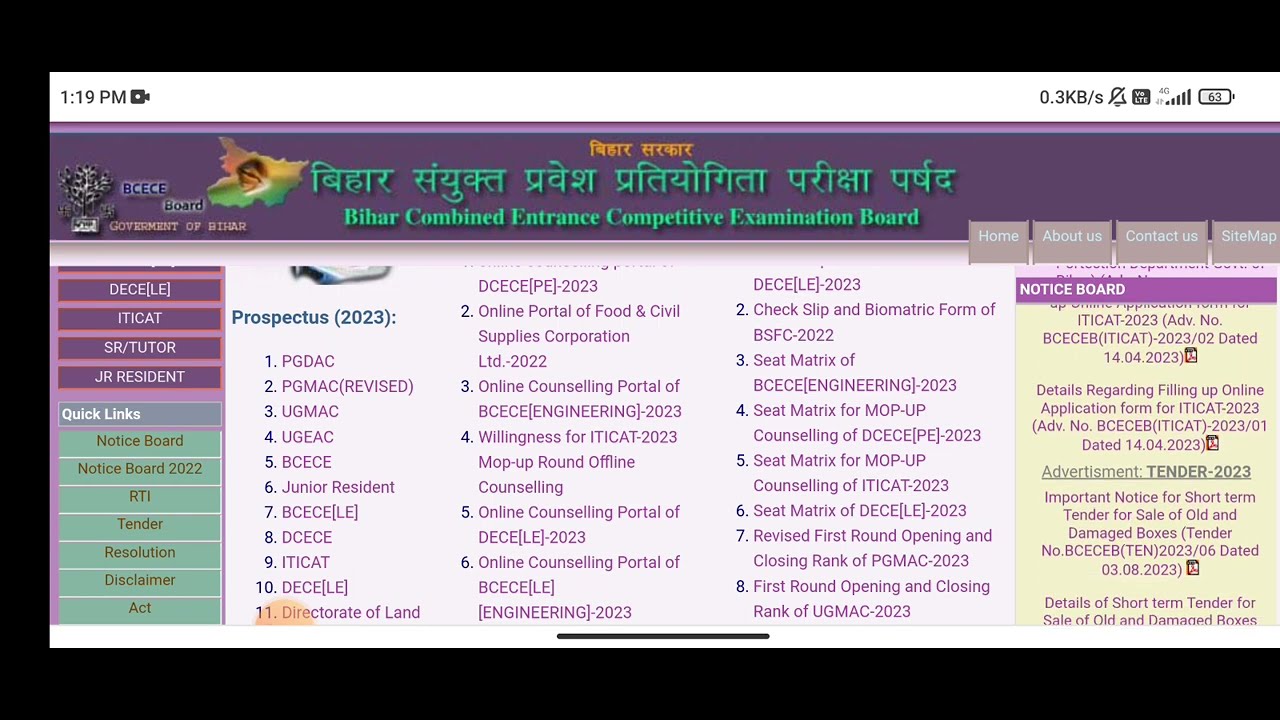The image depicts a computer or phone screen showcasing a foreign-language website. The top section features a white banner with a black border on the left, top, and bottom edges. The top-left corner displays "1:19 PM" alongside a camera icon, while the top-right corner shows "0.3 KBs," a bell icon with a line through it, various other figures, and a battery at 63% charge. Directly below is a purple banner with text in a foreign language. Prominently, in green text, it reads "Bihar Combined Entrance Competitive Examination Board." Beneath this are navigational tabs labeled "About Us," "Home," and "Contact Us." The left side of the screen contains a purple and green sidebar listing "Quick Links," "Notice Board," "Notice Board 2022," "RTI," "Tender," "Resolution," "Disclaimer," and "Act." In the central part of the screen, the title "Prospectus 2023" appears, followed by a detailed list numbered 1 to 11, with additional numbers 2 to 6 in the middle and 2 to 8 on the right. A "Notice Board" section with more information is also present on the right side of the image.